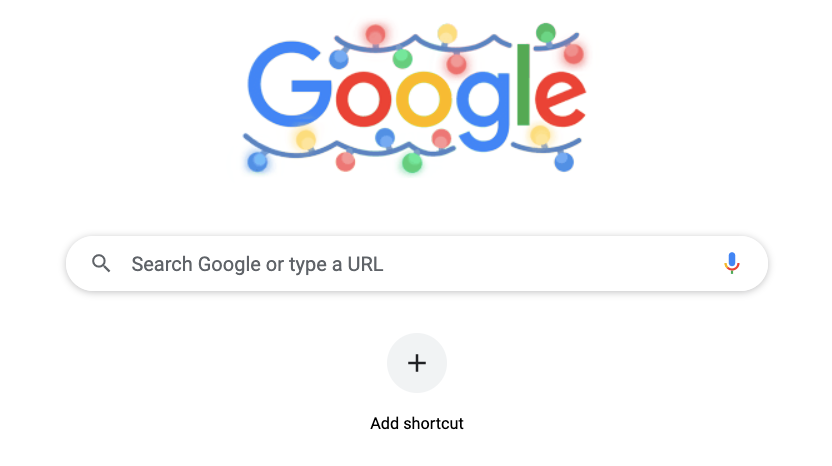The image is a screenshot of the Google search website adorned with festive Christmas lights. At the center top of the page is the iconic Google logo, each letter colored distinctively: the 'G' is blue, 'o' is red, the second 'o' is yellow, 'g' is blue, 'l' is green, and 'e' is red, all in a bold font. Above and below the logo are strings of Christmas lights. The top string features bulbs in the sequence: blue, red, green, yellow, red, green, red, mimicking the colors of the Google logo. The bottom string displays bulbs in the order: blue, yellow, red, blue, green, red, yellow, red.

Beneath the festive logo is the search bar in a smooth rectangular shape. Inside the search bar, the placeholder text reads "Search Google or type a URL" in a light black font. To the left within the bar is a magnifying glass icon, and to the right is a colorful microphone icon with blue, red, and green hues. Directly below the search bar, centered at the bottom of the image, is the text "Add shortcut" accompanied by a small plus symbol above it.